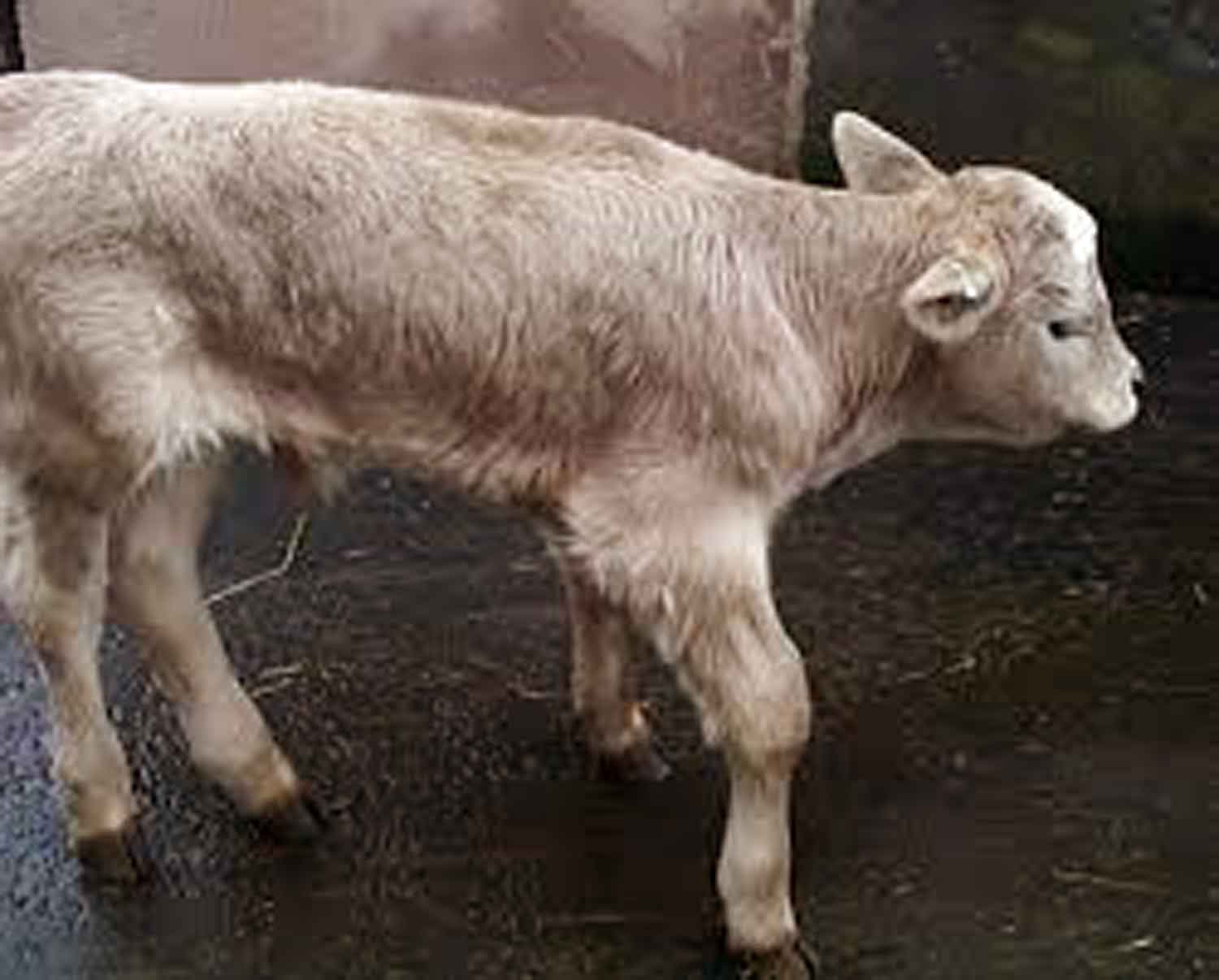The image prominently features a baby calf, appearing somewhat thin and in distress, with long, light brownish-white fur and darker spots. Facing the right, its black eye, half of its black nose, and both slightly lowered ears are visible. The calf stands on a wet, possibly muddy or concrete surface with scattered hay or grass, making its black hooves clearly noticeable. The background is blurry and dark, suggesting a damp environment. In the bottom right corner, there's a light and dark brown square-shaped object. The overall setting and the calf’s posture suggest it might be in a challenging or uncomfortable situation.